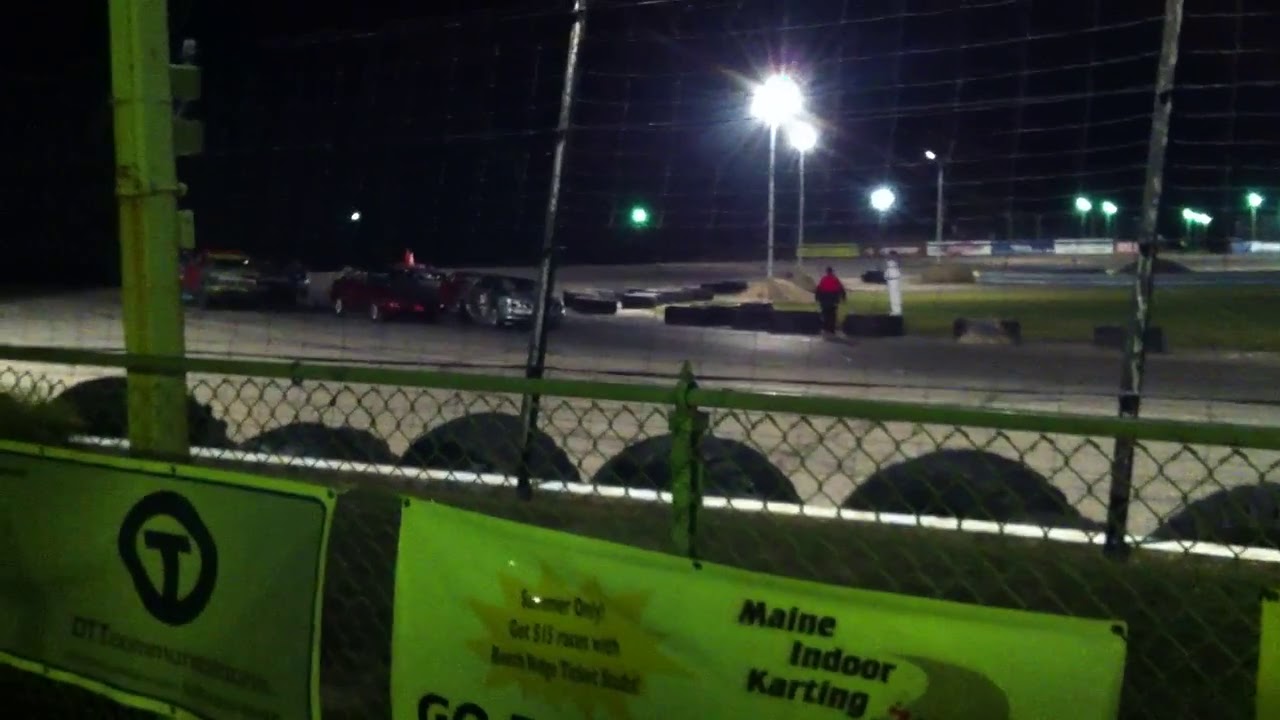This nighttime photograph captures an outdoor go-kart track, viewed from behind a chain-link fence adorned with green banners and advertisements, including one partially reading "main indoor karting" and another featuring a "DT" logo. Positioned right at the front, the fence precedes a row of tires acting as barriers on the opposite side. The well-lit track itself has several regular cars lined up, not go-karts, with the clean, green-tinted surface illuminated by tall floodlights. A solitary person, identifiable by a red and black jacket, is seen walking away on the far side of the track. No other individuals are visible in the scene.